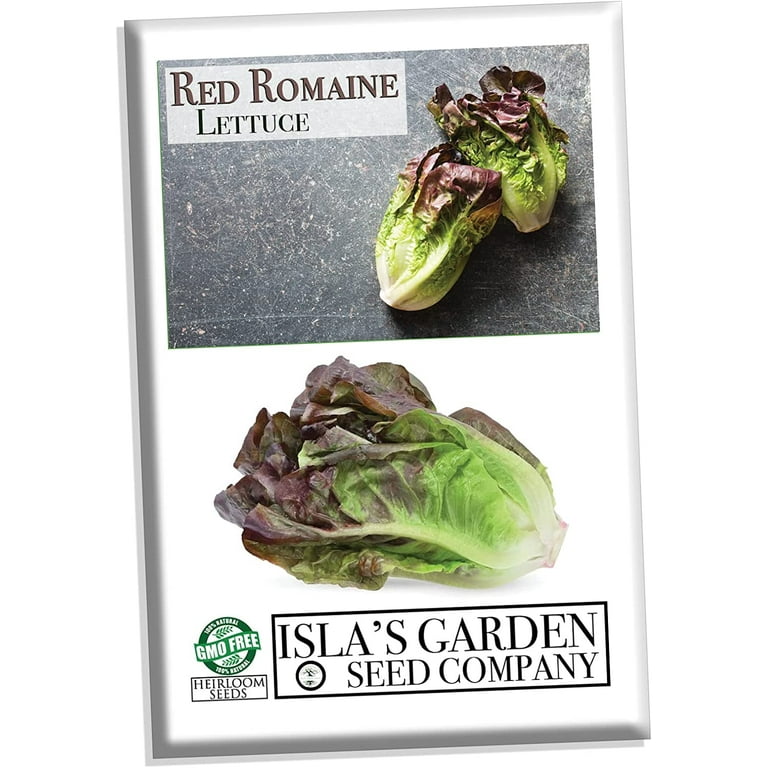This is an image of a seed packet from Isla's Garden Seed Company, showcasing their Red Romaine Lettuce. The packet features a predominantly white background with two images of the lettuce. 

The top image, set against a gray speckled surface, displays two clusters of deep red romaine lettuce, labeled as "Red Romaine Lettuce." 

The bottom half of the packet highlights a larger, single head of the same lettuce on a plain white background. To the left of this larger lettuce image, there is a green symbol indicating "GMO-free," and below it, in a smaller boxed image, it says "Heirloom Seeds." At the very bottom, it is clearly labeled "Isla's Garden Seed Company." 

This detailed presentation, complete with descriptors like "GMO-free," "100% natural," and "Heirloom Seeds," suggests that this is a seed packet meant to advertise and sell heirloom, GMO-free red romaine lettuce seeds.